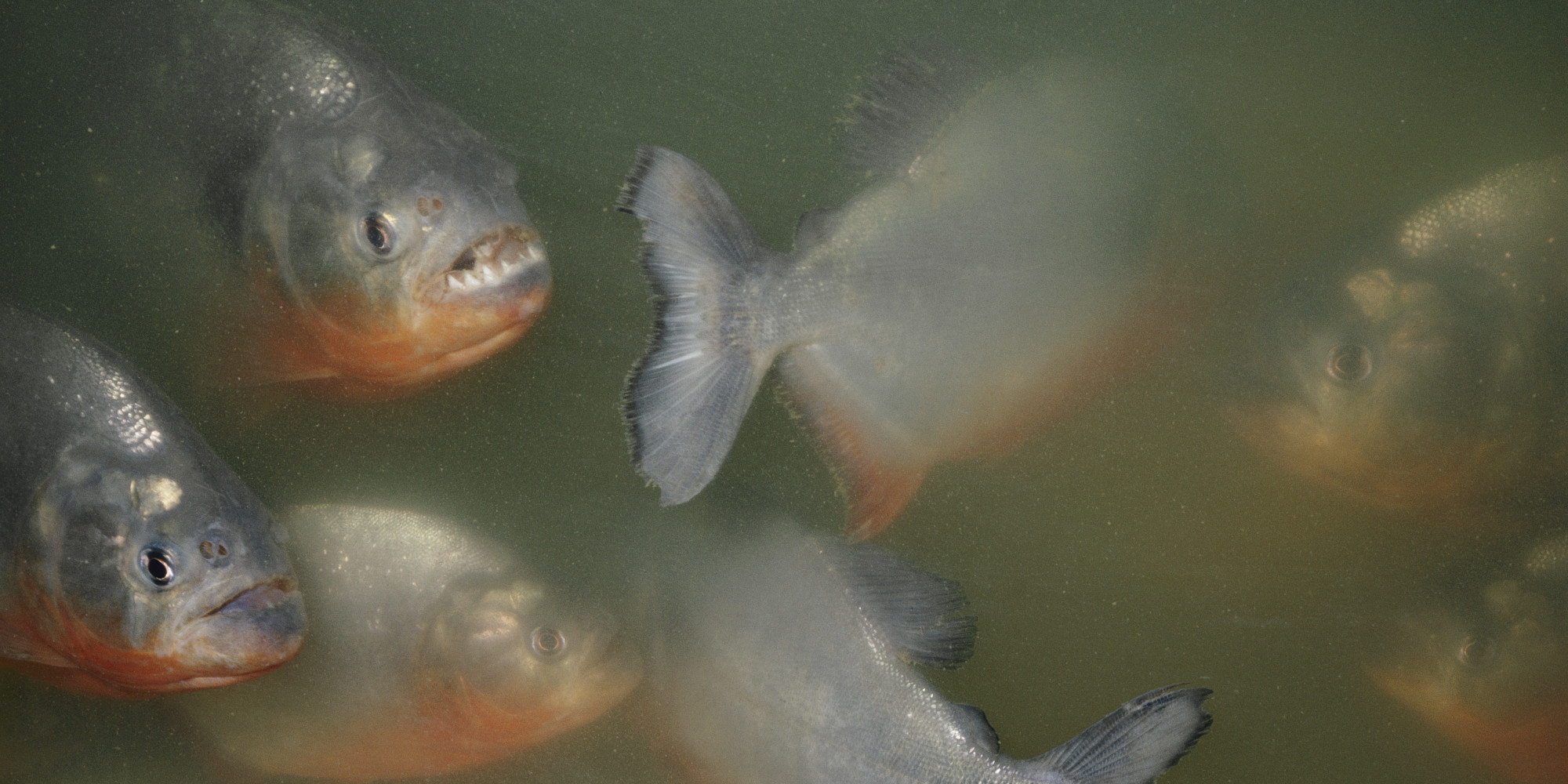In the murky, dark green water of the image, there is a school of seven medium-sized, silver-gray fish, each featuring red or orange hues on their bellies. The two most distinct fish are on the left side of the image, swimming towards the viewer. One of these fish, positioned at the top, has its mouth open, displaying a row of sharp, jagged teeth, while the other has its mouth closed. Among the other fish, two appear to be swimming away, showing only their backs and back fins. Additionally, three fish provide a side view with black eyes, also facing towards the left of the image. Despite the murkiness of the water, the details of the fish — including their slightly elevated mouths and side-placed eyes — are visible, emphasizing the eerie underwater setting.